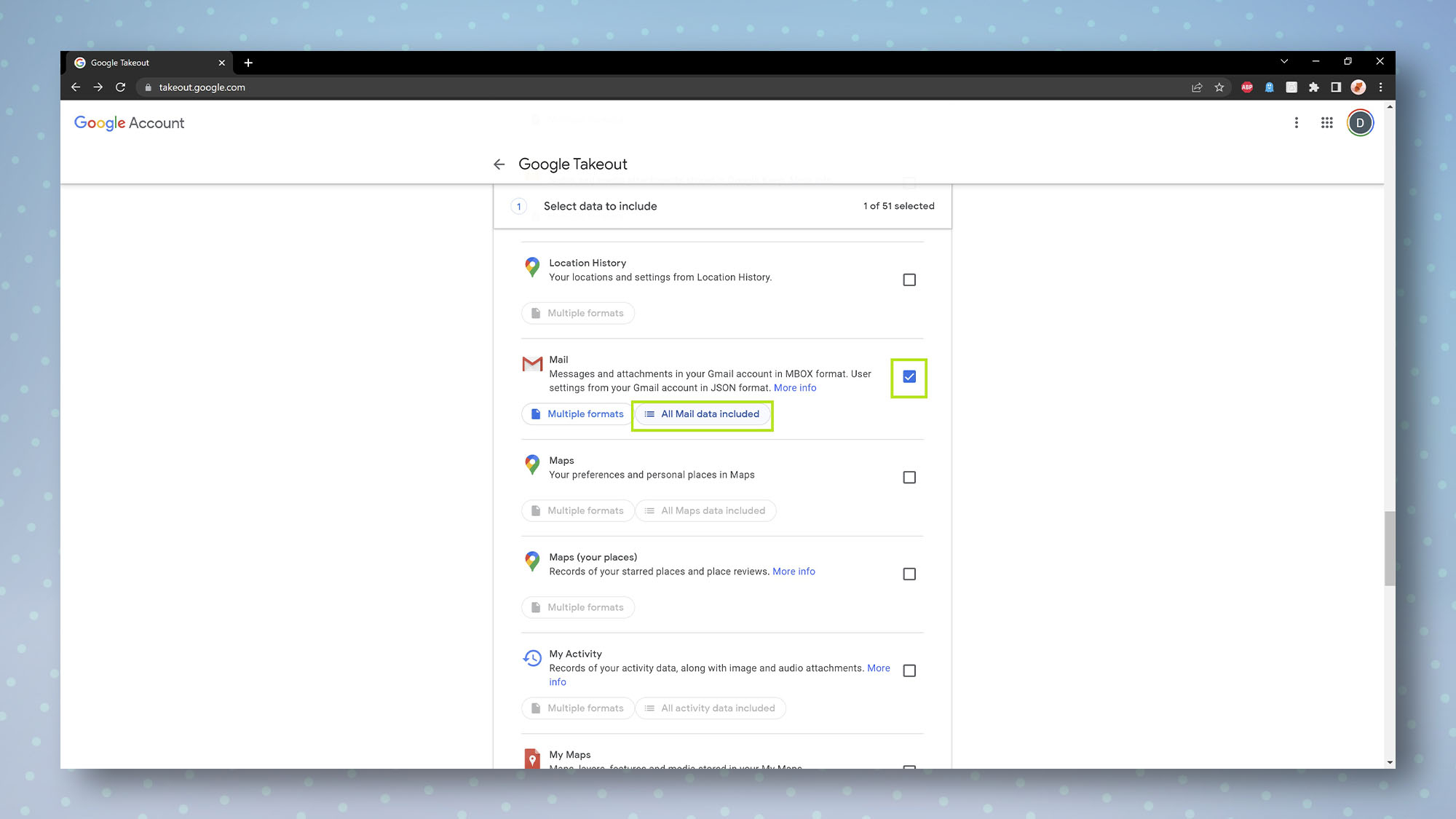The screenshot captures a portion of a web browser displaying the Google Takeout page, accessible at takeout.google.com. The browser tab is labeled "Google Takeout." In the top left corner of the webpage, the "Google Account" label is visible, while the top right corner features a menu icon and a user account button.

The central section of the page is titled "Google Takeout," accompanied by the instruction "Select data to include." At this moment, only one out of 51 available data selections is chosen.

Immediately visible on the list are several options for data export, beginning with "Location History," followed by "Mail." The Mail section provides further details: it includes "Messages and attachments in your Gmail account in inbox format" and "User settings from your Gmail account in JSON format." It also states "Multiple formats and all mail data included," next to a checkbox. This checkbox, alongside the text "all mail data included," is highlighted with a yellow outline. The Mail option is the only selection with its checkbox marked.

Subsequent items in the list include "Maps," "Maps (your places)," "My Activity," and "My Maps," each accompanied by their respective unselected checkboxes.